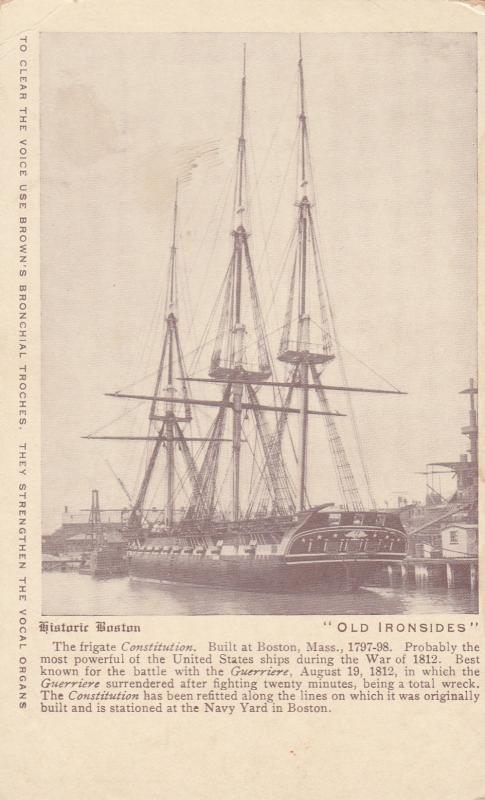The image depicted is an aged newspaper clipping from the early 1800s, specifically 1812, showcasing an illustration of the historic frigate, the USS Constitution, famously nicknamed "Old Ironsides." The clipping’s text is somewhat difficult to decipher due to its age and small font size, but it provides a detailed account of the ship’s significance. Built in Boston, Massachusetts between 1797 and 1798, the Constitution was one of the most formidable ships in the United States Navy during the War of 1812. The text highlights the ship’s notable engagement with the British frigate Guerriere on August 19, 1812, where the Guerriere surrendered after merely 20 minutes of combat, ending as a total wreck. The ship, depicted with its three masts bare of sails, stands as a testament to its durability and the American naval prowess of its era.